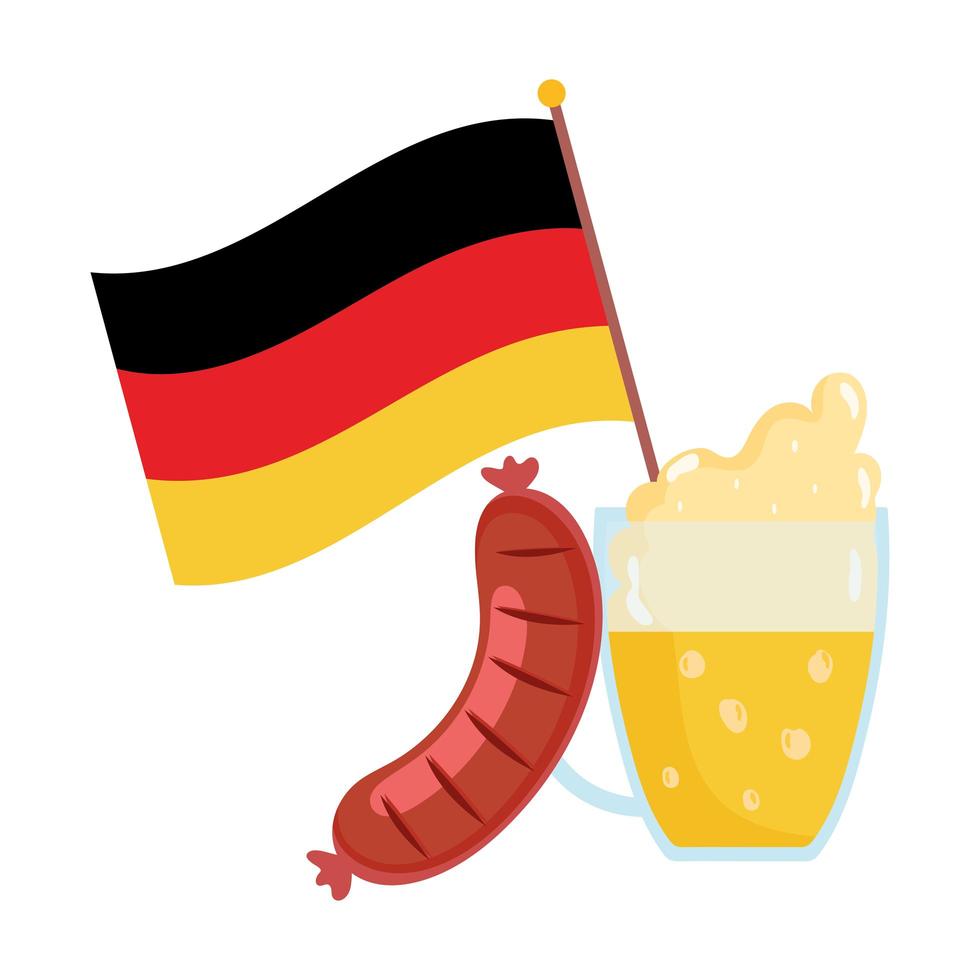This is a vector-style advertising image, resembling clip art, showcasing a German Oktoberfest theme. At the center, there's a clear glass with a handle, reminiscent of a coffee mug, filled with a golden, amber-colored liquid with white frothy bubbles and foam on top, indicating it is beer. A bratwurst sausage, characterized by its reddish-brown color and twisted ends, is curved and propped against the beer glass. Emerging from the glass is a German flag, featuring black, red, and gold horizontal stripes. The background is plain white, enhancing the simplicity and focus on the elements. Overall, the image emphasizes traditional German symbols, likely to evoke the festive atmosphere of Oktoberfest.